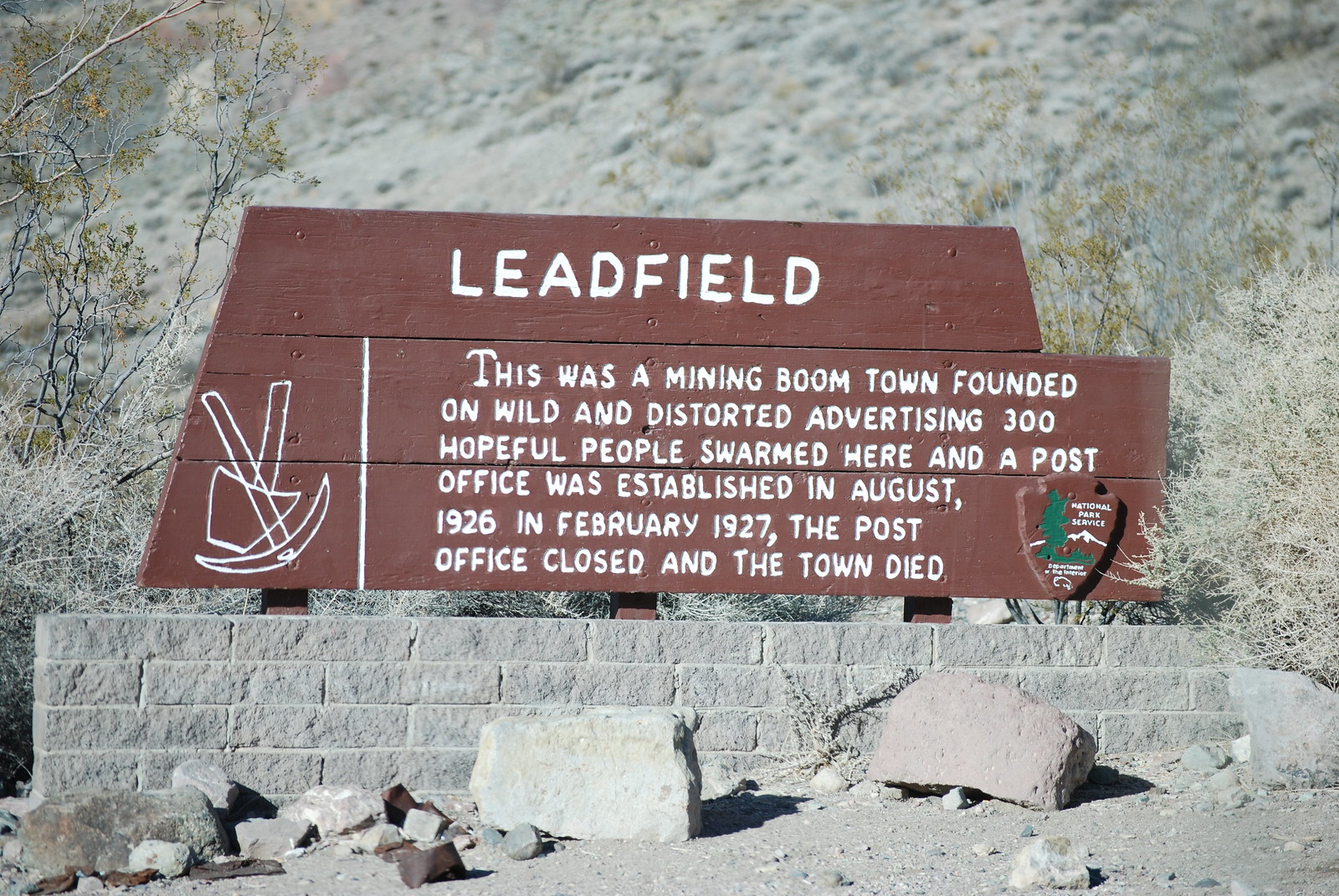The image shows a historic site marked by a brown wooden sign, prominently placed atop a small stone wall built from white cinder block-like bricks, with various crumbled rocks scattered at its base. The sign details the history of Leadfield, a mining boom town that rose quickly from wild and distorted advertising, drawing 300 hopeful residents who established a post office in August 1926. By February 1927, the post office closed, marking the town's demise. The sign features a hand-painted illustration of a shovel and pickaxe on the left side and is topped with the word "Leadfield" in white letters. In the bottom right corner, a plaque bears the National Park Service emblem. The background reveals a rocky hillside with sparse, grayish brush and a few scattered trees, suggesting a desert-like environment.